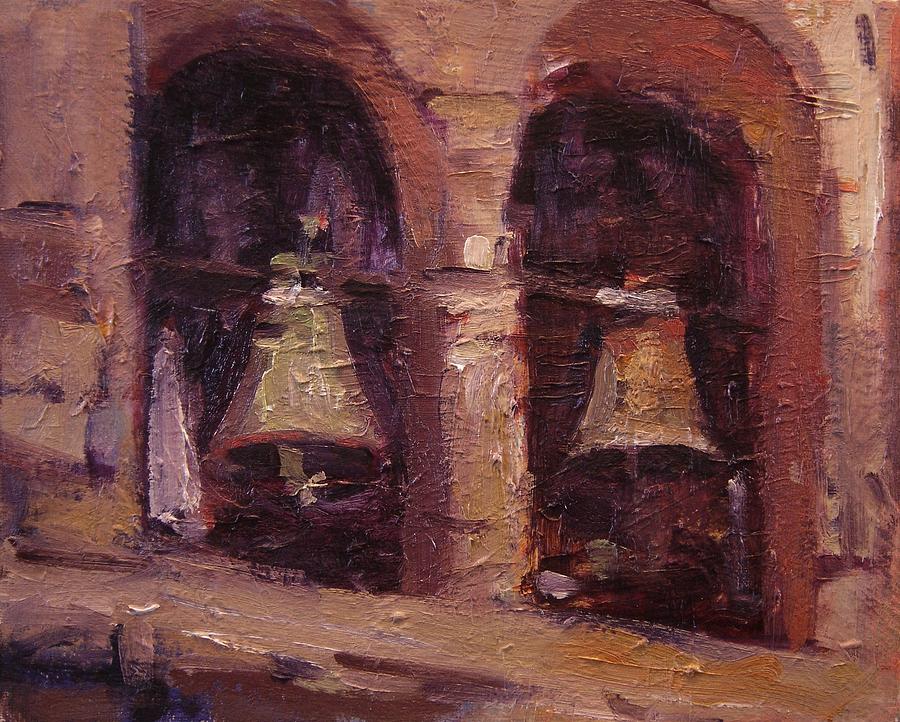This detailed oil-based painting by Meryl Dressley depicts a decaying, stone church building with two prominent bell tower windows. The composition offers a close-up view that emphasizes the heavy application of paint and the rich texture, particularly in the areas showcasing shades of brown, orange, yellow, and hints of green and gold. The structure appears old and worn, with dark recesses suggesting an ancient, possibly abandoned church. Inside the windows, the bells are mounted on a wooden support; one bell is greenish, while the other glows a golden hue. A wooden plank extends across to reinforce their support. Intricate details include a white cloth hanging to the left of one bell and a small pergola visible just inside the window. The painstakingly crafted image conveys the sense of looking up at the bells, capturing the essence of their central position within the worn brick framework of this historical edifice.